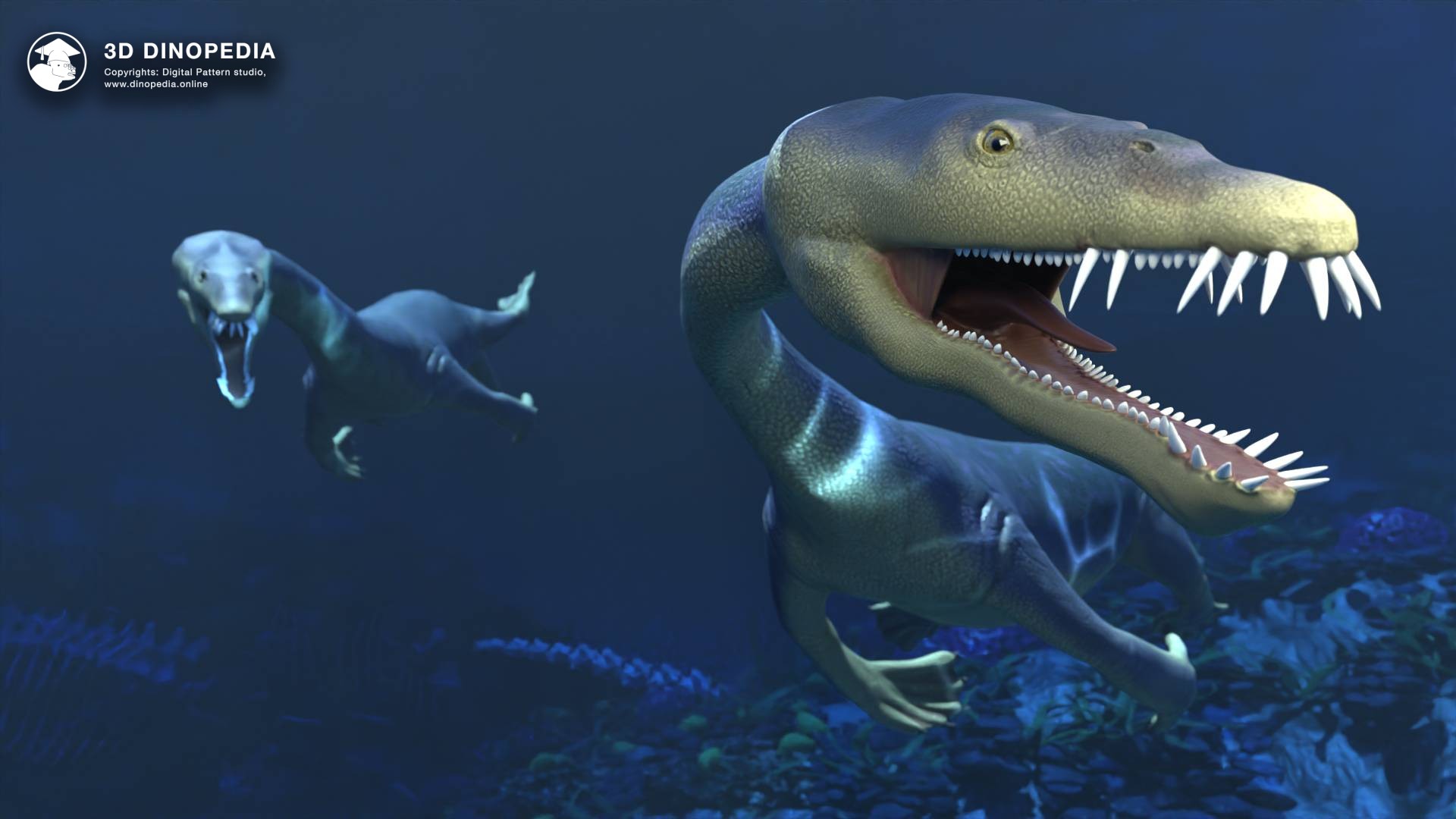The image is a detailed 3D render from the "3D Dino-Pedia," evident by the logo and the text "3D Dino-Pedia" in the top left corner, with additional copyright details from Digital Pattern Studio (www.dinopedia.com). The scene appears to be underwater, featuring two dinosaurs with elongated necks and snouts similar to those of alligators, filled with sharp, white teeth. The larger dinosaur, prominently displayed on the right, displays a long tail, fins instead of traditional legs, and wide open eyes, with a light illuminating its head. Its front fins appear longer than its back fins. The smaller, similar dinosaur is depicted further away on the left side of the image. The color palette includes dark and light blues representing the water, with the dinosaurs themselves in shades of green, accented with tans and creams on their underbellies, and a dark reddish hue inside their mouths.